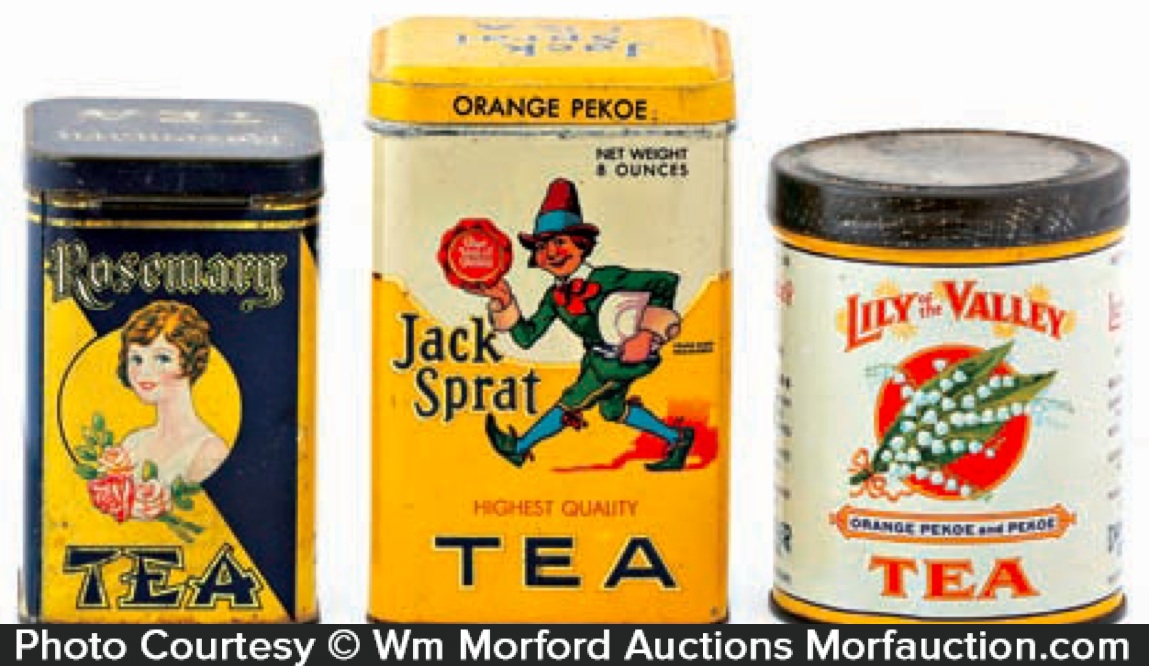The image features three vintage tea containers set against a white background. On the left, there's a navy blue rectangular tin with gold accents. The front displays a yellow and navy split background, with the word "Rosemary" in navy blue text on the yellow half, and "Tea" beneath it in smaller blue letters. In the center of the tin is a circular illustration of a smiling woman with short brown hair, pink skin, and pink flowers in her hair, drawn in a cartoon style reminiscent of the 1920s era.

The middle container is also rectangular and sports an orangish-yellow hue. The top half of its front is beige while the bottom half continues the orangish-yellow color. It prominently features the label "Jack Sprat" along with the text "Highest Quality Tea." The central illustration is of a cartoonish young man resembling a pilgrim, wearing a brown hat, a green jacket, a red bow, and blue socks pulled up to his knees, smiling amid the red circle adornment.

On the right is a cylindrical tin with a white body and a brown top. It features "Lily of the Valley" in red text, along with "Orange Pico and Pekoe Tea." Dominating the front is a red circle enclosing an image of the Lily of the Valley plant, illustrated with white bell-shaped flowers against green leaves. At the bottom, a black stripe with white lettering reads, "Photo courtesy copyright W.M. Morford Auctions. MorfordAuction.com."

The array of colors includes dark blues, yellows, reds, greens, orangish yellows, pinks, and navy, all contributing to the distinct vintage charm of these tea containers.